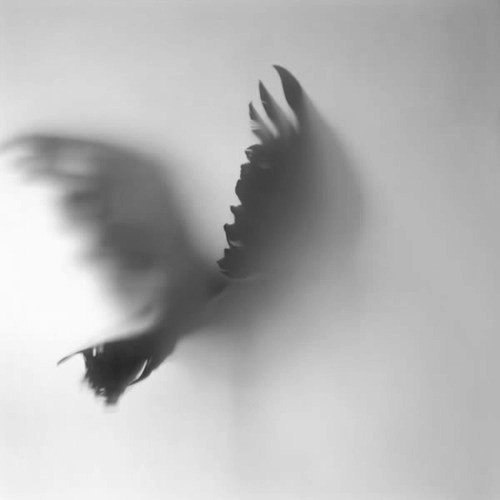In a black and white photograph shrouded in a haze and mist, an airborne bird is captured in mid-flight, moving away from the viewer and deeper into a dense fog. The bird's dark silhouette, which appears nearly black but is partially obscured by the cloud, is discernable mainly by its outstretched wings and distinct tail feathers. The background is a diffuse wash of white and gray, adding to the photo's ethereal, blurred quality. The right wing, more defined and closer to the camera, contrasts sharply with the left wing, which melds into the fog, rendering it softer and more gray. The intricate details of the individual feathers on both the wings and tail are visible, even as the rest of the bird's body, particularly the head, remains obscured. The bird's wings seem to be positioned as though flapping upwards, centered in the image yet predominantly leaning toward the left side, creating a dynamic yet ghostly visual of avian motion through the mist.